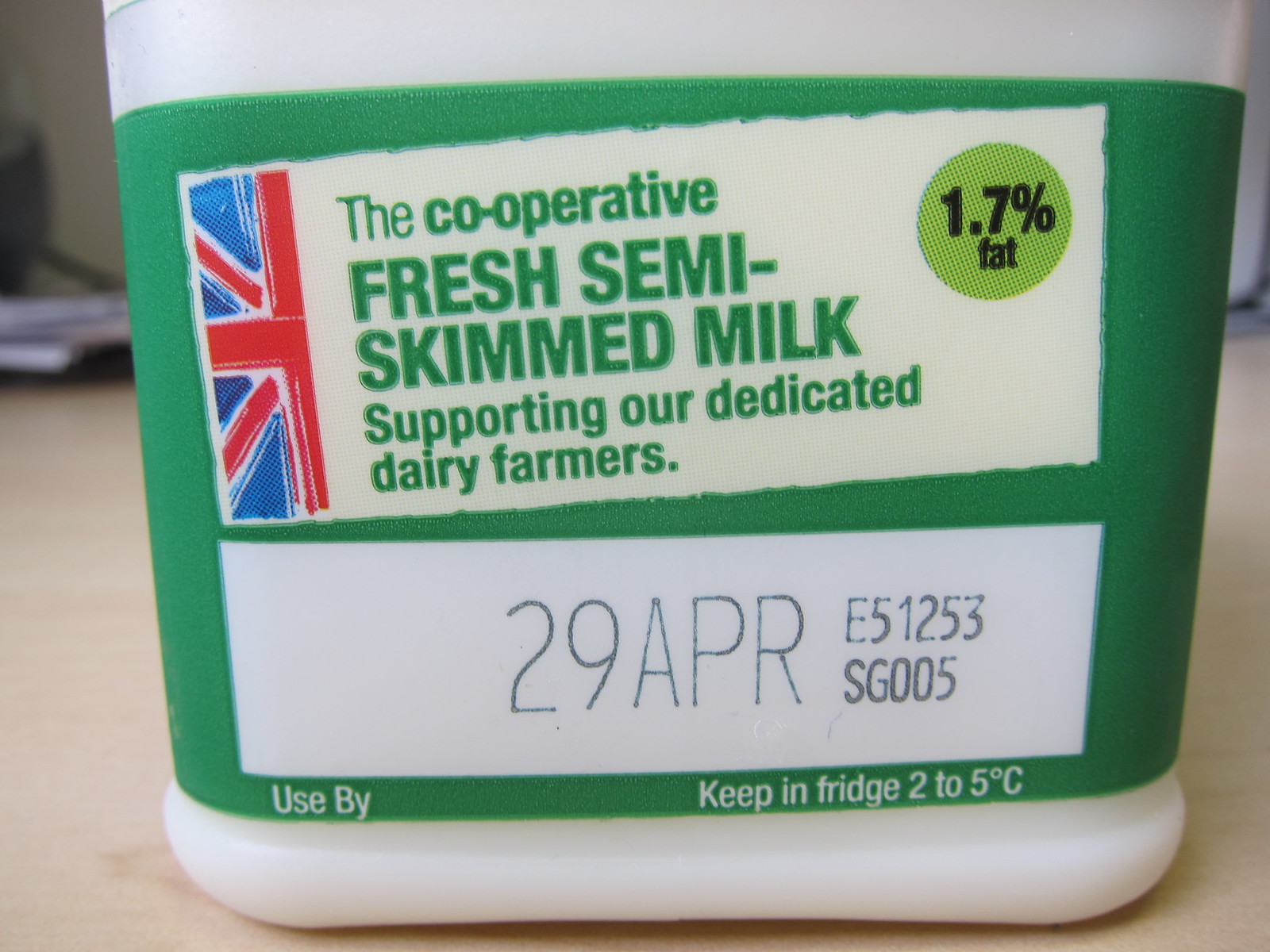The image is a close-up photograph of a white, square plastic bottle of milk, positioned on a light tan-colored table, taken indoors. The bottle prominently features a green and white label encircling its lower half. On the left side of the label is a partial depiction of the British flag, which appears painted. Adjacent to the flag, in green text on a white background, are the words: "The Cooperative Fresh Semi-Skimmed Milk, supporting our dedicated dairy farmers." To the upper right of this text is a green bubble that reads "1.7% fat" in black font. Below this bubble, another white rectangle contains an expiration date: "29 APR," followed by a series of numbers "E51253SG005." Further down on the green label, in white text, are the instructions: "Use by" with the expiry date inferred to be the 29th of April, and "Keep in the fridge from 2 to 5 degrees Celsius."